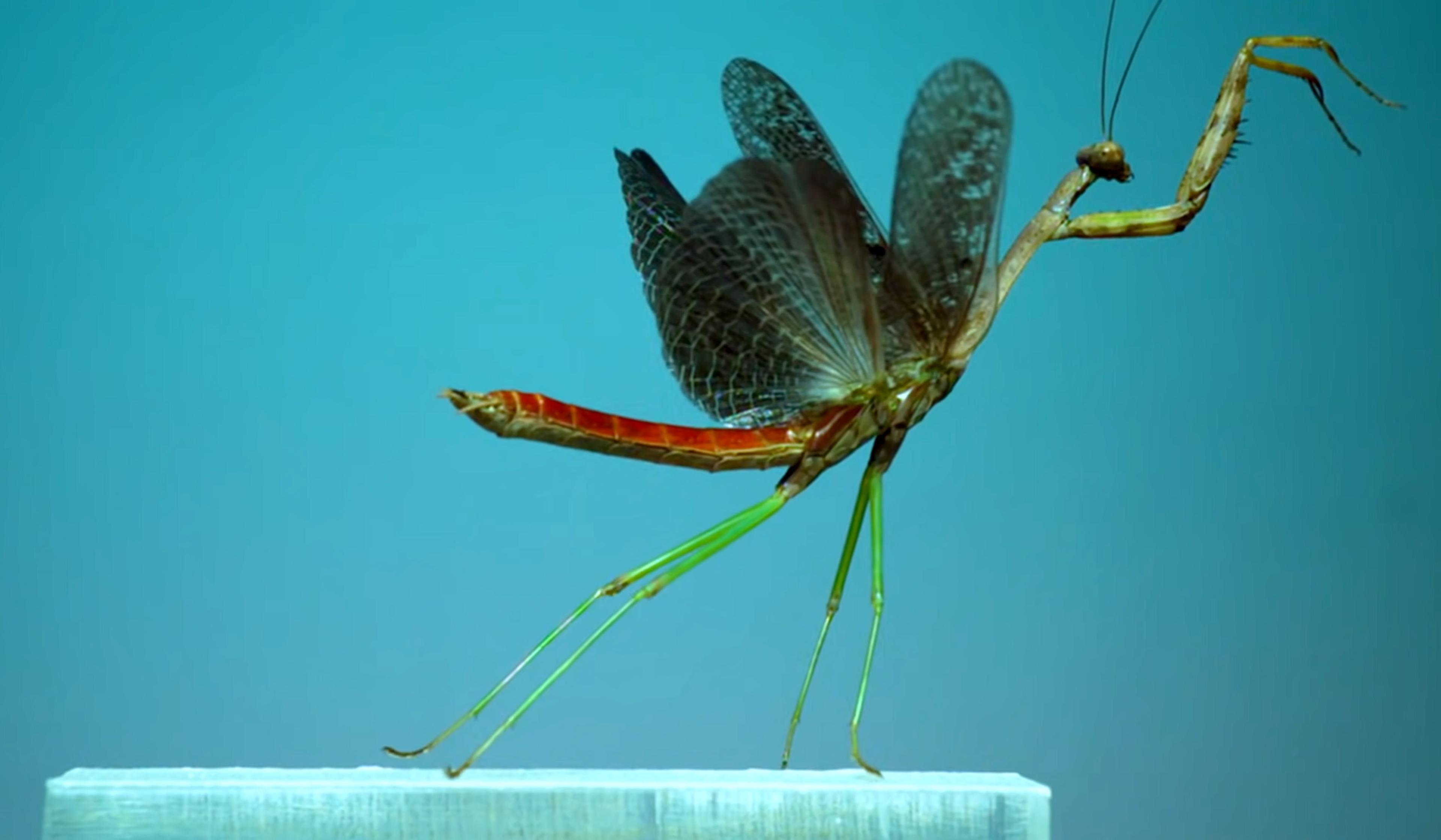This close-up photograph captures a fascinating moment featuring a sleek and slender insect that closely resembles a praying mantis or a katydid. The insect's body is predominantly green, with an elongated, thin structure and extremely long legs. Its small head is crowned with very long antennae. The insect also has a distinctive long tail highlighted by a reddish accent.

One of the most intriguing features of this insect is its set of arms, which are wider and thicker than its body and extend out with finger-like extensions. Dark grayish, possibly black, wings adorn its back, appearing almost as two sets, adding to its intricate appearance. 

The background is a soothing light blue, fading out near the top middle where a lighter light source illuminates the scene. The insect appears to be standing on a white block that could be a piece of ice, vinyl, or plastic. Adding to the complexity, perched or possibly attached to the insect's back is a dragonfly, making the scene even more captivating and mysterious.

Overall, the photograph presents the insect leaning to the right, creating a striking composition. The subtle contrasts and the serene color palette make this image both intriguing and aesthetically pleasing.